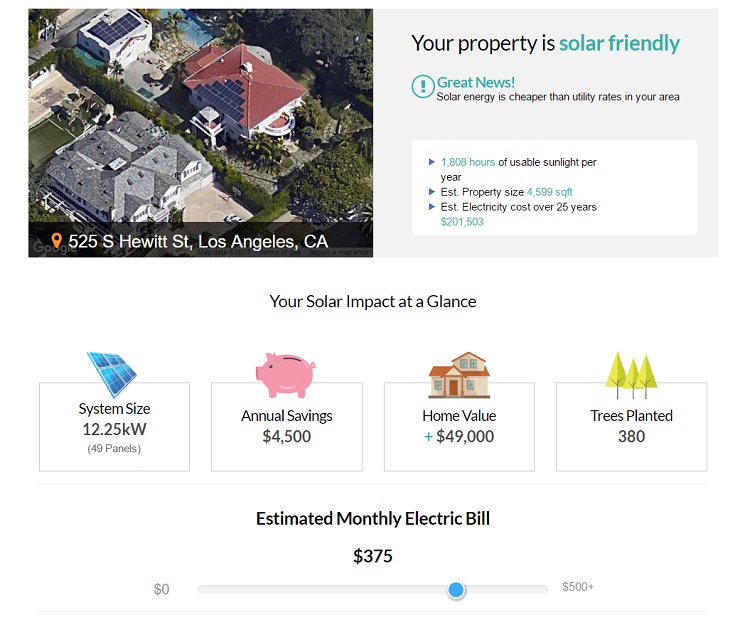Screenshot of a Solar Company Website

The screenshot features a solar panel company's website with detailed information about a property located at 525 South Hewitt Street, Los Angeles, California. On the top-left corner, there is an aerial image showing two houses—one equipped with solar panels and one without. An address pin marks the location at the bottom of the image.

To the right of the photo, a gray box states, "Your property is," followed by the phrase "solar friendly" in teal text. Below this, a teal circle with an exclamation point and the phrase "Great news!" grab attention. In black text, the site highlights that solar energy is more cost-effective than utility rates in the area.

The information is broken down further in a white box below, providing critical data:
- **Usable sunlight per year:** 1,808 hours
- **Estimated property size:** 4,599 square feet
- **Estimated electricity cost over 25 years:** $201,503

Additionally, the section "Your Solar Impact at a Glance" provides a comprehensive overview:
- **System size:** 12.25 kilowatts
- **Number of panels:** 49
- **Annual savings:** $4,500
- **Increase in home value:** $49,000
- **Environmental impact:** Equivalent to planting 380 trees